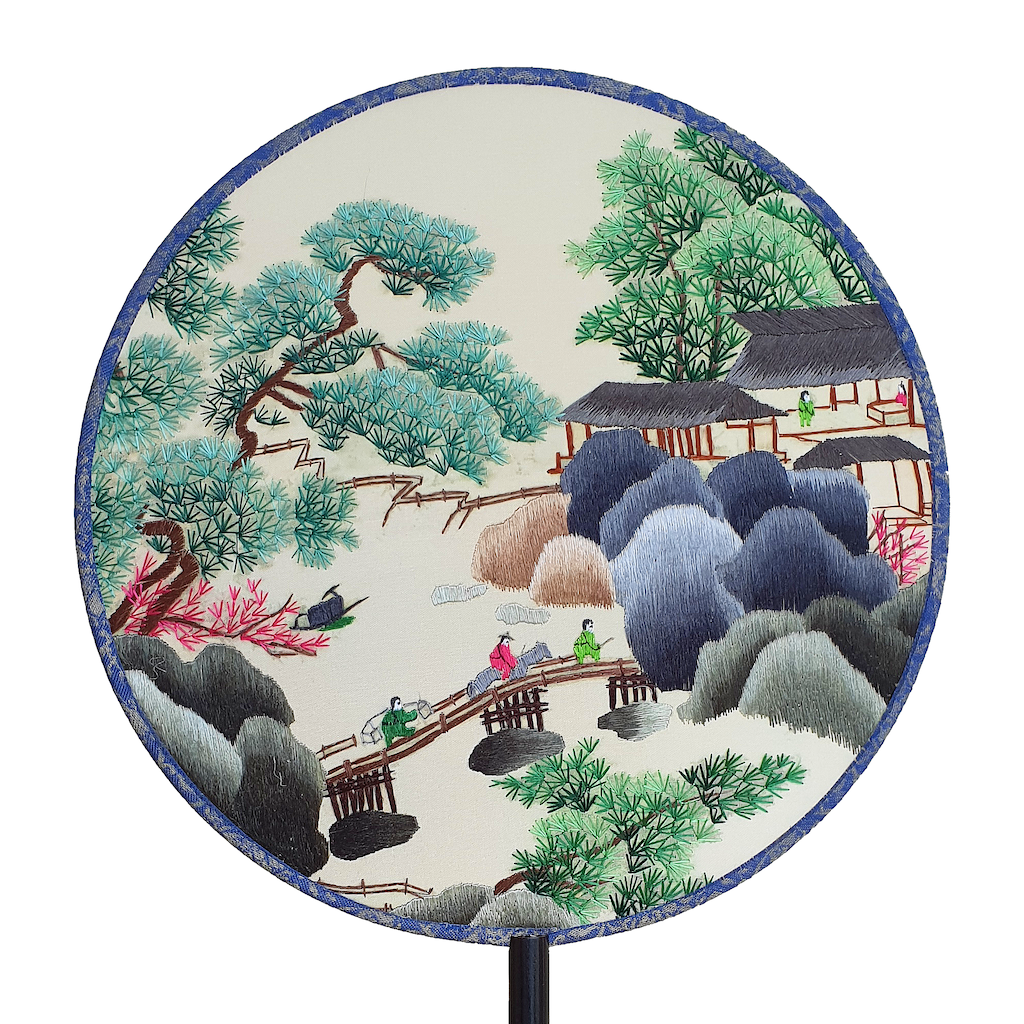This image features a meticulously hand-embroidered, computer-generated depiction of a traditional Chinese silk fan, designed in a circular form with a dark blue border. The artwork portrays an outdoor landscape scene, rendered in a cartoony, simplistic style. On the fan's left side, there's lush greenery with light green leaves and a tree with red flowers and a bird perched in a nest. A river flows beneath a wooden bridge supported by three rocks, over which three figures are crossing. 

The individuals include a man with a shoulder harness carrying items, a person in a green robe, and another in a red robe and conical hat riding a blue horse; the latter figure appears to also have a sword, indicated by the visible handle. The bridge leads to a land adorned with blue, gray, and brown bushes. 

Beyond the bushes lies a trio of primitive pavilions, two of which have blue gable roofs with brown beams, their interiors visible through open walls. A person in a green robe is seen sitting on a tatami mat within one of the pavilions. Above the buildings, more green trees with needle-like leaves and brown branches extend to the top right section of the composition. The fan artistically amalgamates detailed elements and a vivid color palette to create this picturesque Asian landscape scene.